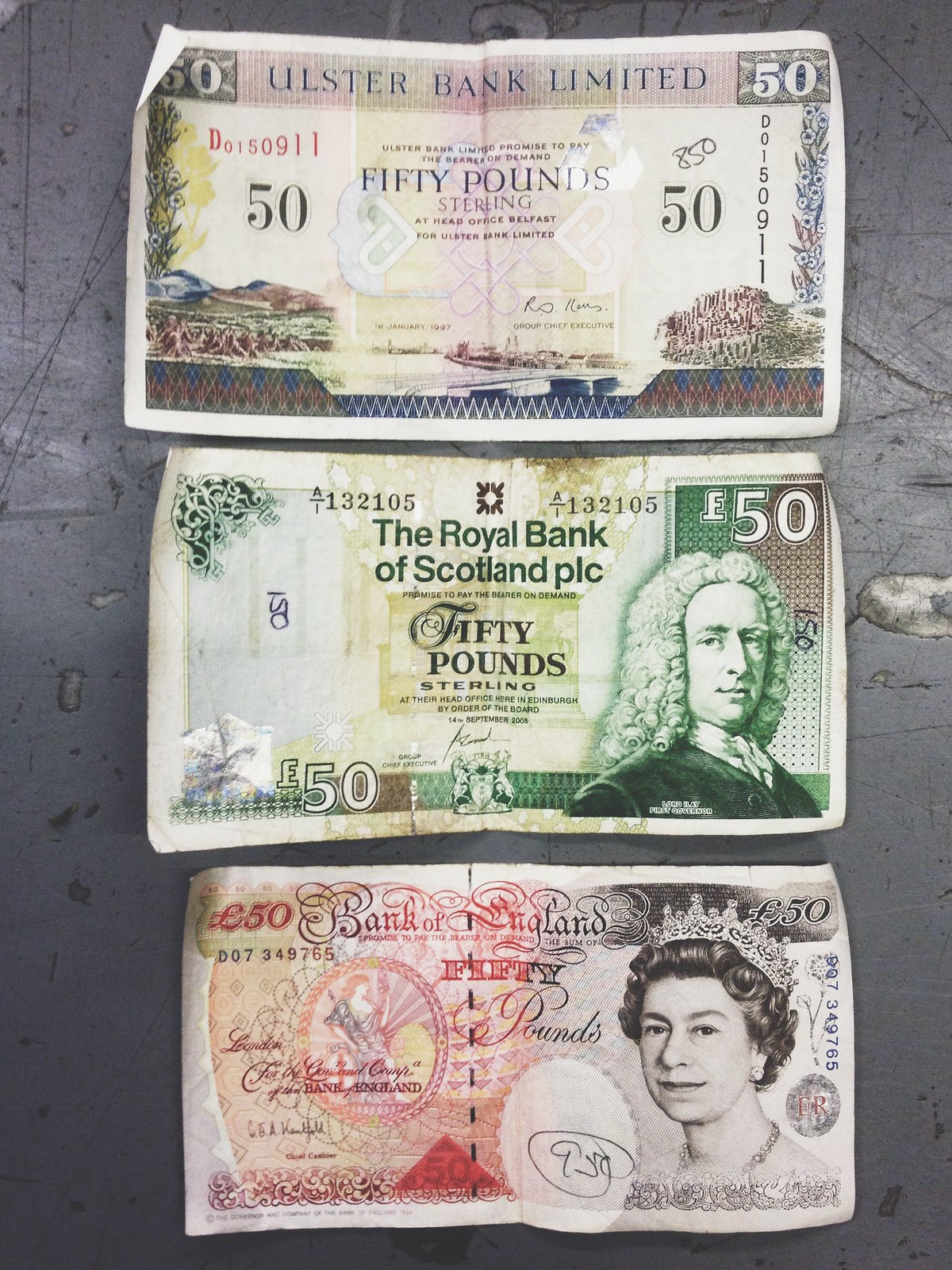In this image, three distinct banknotes are meticulously arranged on a heavily scratched and dented gray metal surface. The topmost note is a 50-pound sterling from Ulster Bank Limited, prominently featuring the institution's name and the promise to pay the bearer 50 pounds sterling at their head office in Belfast. The note is adorned with a scenic landscape, showcasing hills and foliage in hues of blue, pink, and white, and is dated January 1997, signed by the Chief Executive.

The middle banknote also represents a 50-pound sterling, issued by the Royal Bank of Scotland PLC. This note includes a historical figure, Lord Ilay, depicted in traditional attire with a powdered wig, indicating the note's authenticity and heritage. The date on this note is September 14, 2008.

The bottom note, again a 50-pound sterling, is issued by the Bank of England. It prominently features an image of Queen Elizabeth II on the right side and includes an artistic depiction of a goddess figure on the left. Each note is distinctly marked with the number "50" denoting its denomination, and collectively, they highlight the rich historical and cultural tapestry embedded in UK currency.